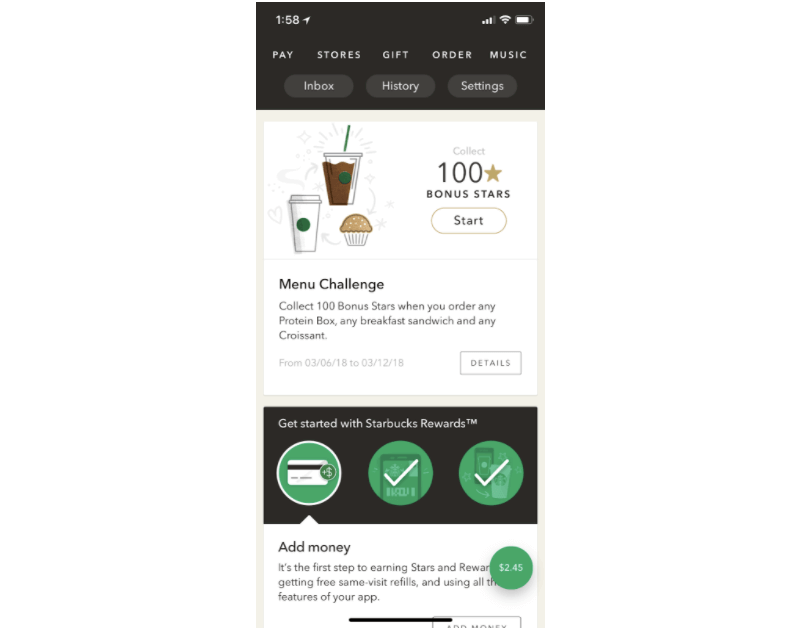This is a detailed screenshot of a smartphone screen. The time displayed is 1:58 PM, and the battery icon shows that the battery is almost fully charged. Two internet icons are visible on the status bar. The main content of the screenshot is the Starbucks app, showcasing several user interface elements.

At the top of the app, five tabs are visible: "Pay," "Stores," "Gift," "Order," and "Music." Below these tabs are three more options: "Inbox," "History," and "Settings." Further down, there's a white box featuring animated drawings of a Starbucks iced coffee, a coffee cup with a green circle in the center, and a muffin. Arrows connect these items in a circular pattern.

To the right of the animated drawings, there is text that reads: "Collect 100 stars, bonus stars, and start. Menu Challenge. Collect 100 bonus stars when you order any protein box, any breakfast sandwich, and any croissant." The promotion is valid from March 6, 2018, to March 12, 2018. There is also a box labeled "Details."

At the bottom of the screen, a black box features the text "Get started with Starbucks Rewards." It includes three green circles representing steps in the rewards process. The first circle, depicting a credit card, has an upward caret and an accompanying description: "Add money. It’s the first step to earning stars and rewards, etc." The next two circles have green check marks, indicating these steps have already been completed.

Finally, at the bottom-right corner of the screen, a green circle displays the current balance of $2.45.